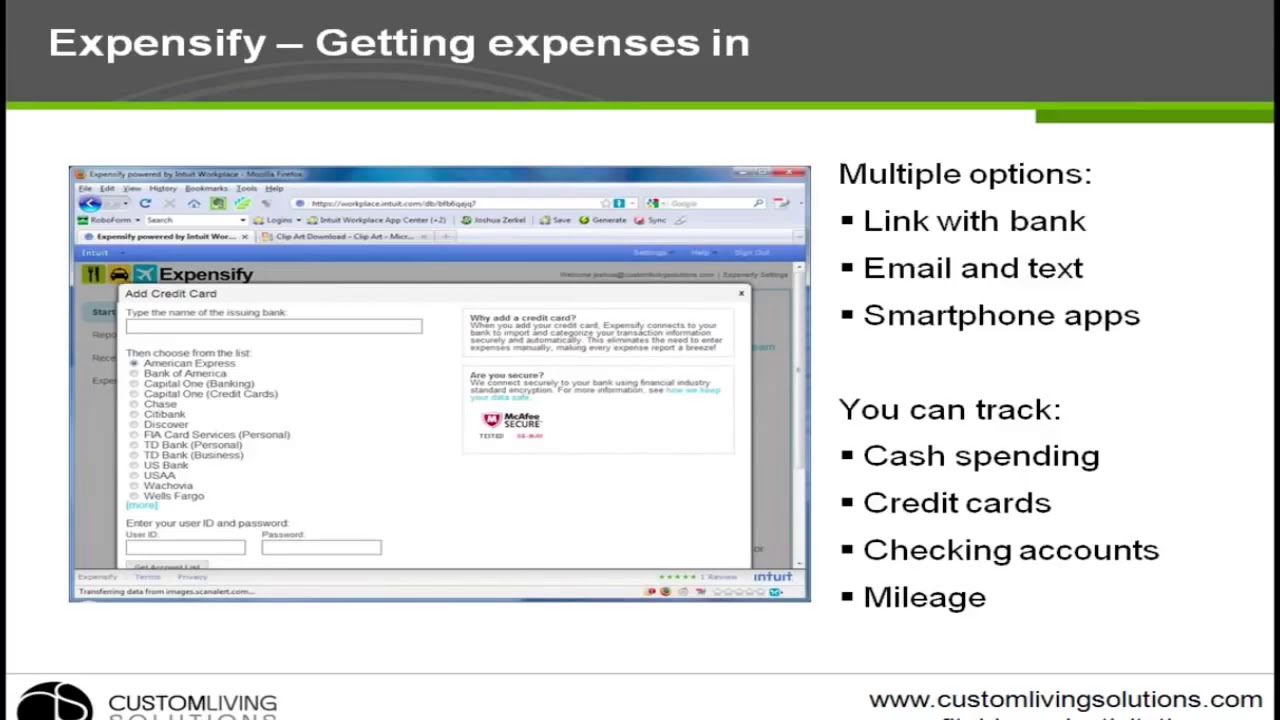The image appears to be a slide from a PowerPoint presentation showcasing the software program Expensify by CustomLivingSolutions.com. At the top of the slide, there is a dark gray bar stretching horizontally across the slide with a green border beneath it. The white text on the gray bar reads, "Expensify: Getting Expenses In." 

On the left side of the slide, there is a screenshot depicting where users can add a credit card with fields to type in the name of an existing bank, along with options to add various banks such as American Express, Bank of America, Capital One, Discover, and Citibank.

On the right side, there are two bullet-point lists. The first list, titled "Multiple Options," includes the options: link with bank, email and text, and smartphone apps. The second list states that users can track cash spending, credit cards, checking accounts, and mileage. 

At the bottom of the slide, the Custom Living Solutions logo is visible on the left, while the URL www.CustomLivingSolutions.com is displayed in black text on the bottom right. The overall background color of the slide is white.